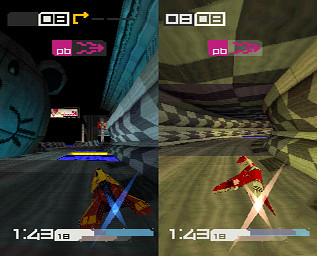The image is a screenshot of a split-screen racing video game, featuring two flying spaceships navigating through distinct yet seemingly interconnected tracks. The left half of the screen showcases a spaceship in the lower right corner, which is beige with blue and gray accents and marked with "143" and "1B". The background here is blue and gray, creating a futuristic atmosphere. Above the ship, we see purple arrows and purple blocks labeled "PB" or "OO" about a quarter down from the top.

On the right side, the spaceship is red and white with a bright yellow taillight, casting a tunnel-like, brightly lit path. The track here features a checkered pattern of gray and black on the floors and walls, and geometric designs on the ceiling in shades of brown and beige. The HUD at the top of the screen is stylized with elements in white, black, purple, and translucent gray. Numbers like "1", "4", "3", and "18" are prominently displayed in white. Both screens show vivid colors including blue, red, yellow, grey, and black, with matching arrows and symbols indicating speed or direction. Overall, the image captures a high-speed, multi-player futuristic racing game with intricate and vividly designed tracks.